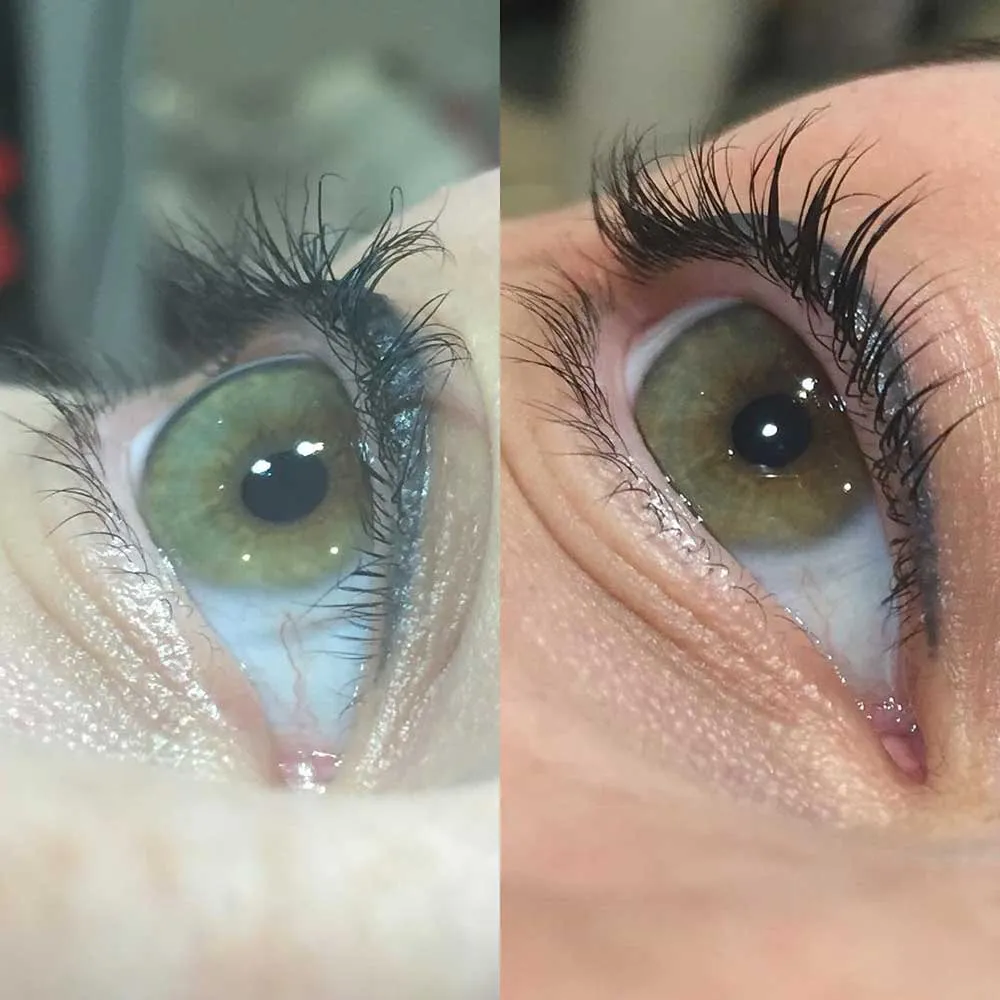This image is a side-by-side comparison of two close-up photographs of a hazel or green eye, likely from the same person. On the left, the image appears lighter, less saturated, and somewhat faded. The eye looks slightly wider open and shows more bloodshot areas in the whites. The skin around this eye is paler, with the photograph exhibiting a generally cloudier quality. On the right, the image is much clearer, with more natural skin tones and a higher level of detail. The eye is similarly hazel or green, framed by defined black eyelashes, and appears less pale and more lifelike than the left. The surrounding flesh on the upper cheek and forehead is visible in both photos, and in both, the background remains blurry and unidentifiable. Overall, the right side is crisp and vibrant, contrasting with the left side's washed-out and foggy appearance.